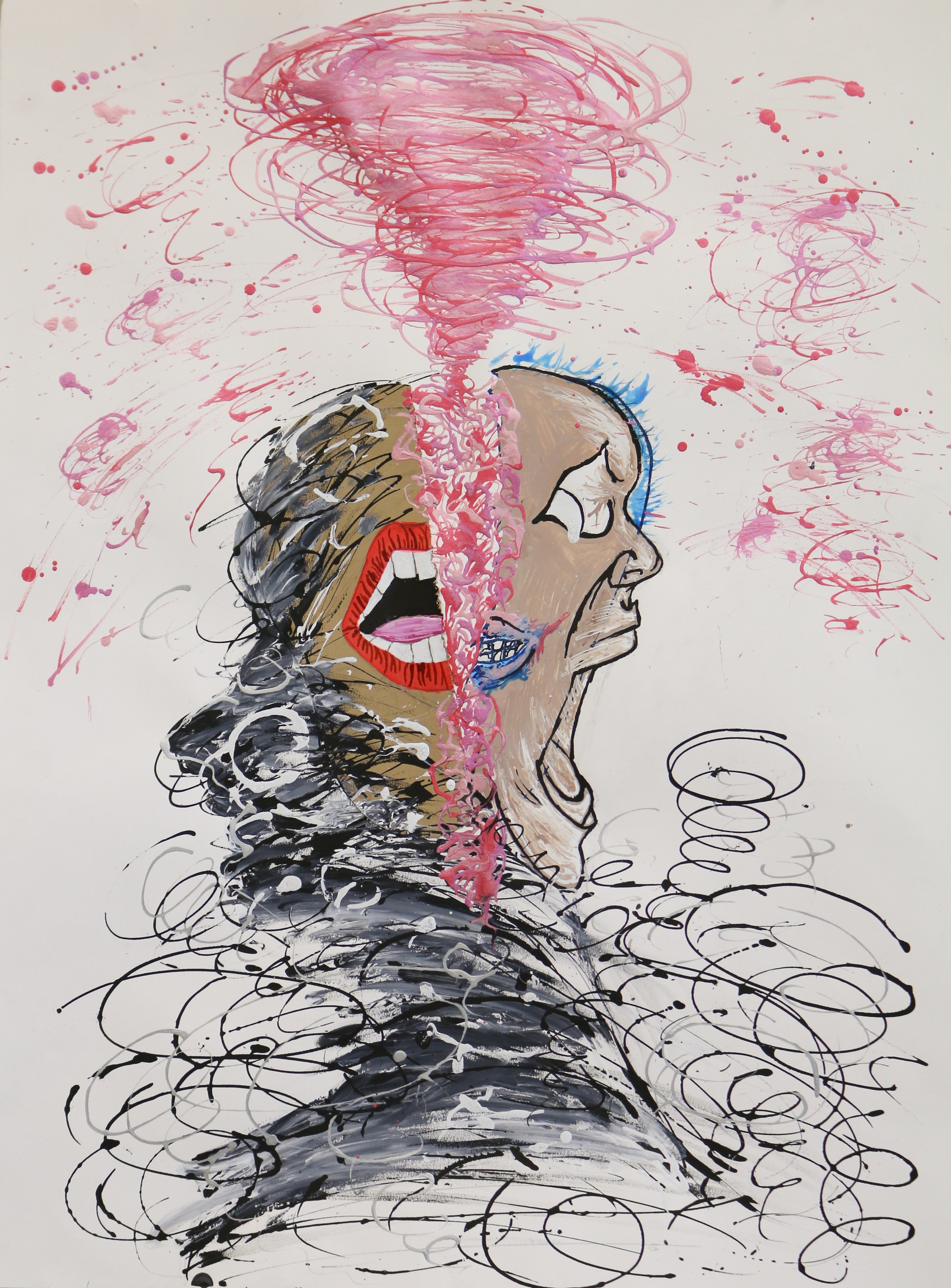This artwork is an intricate and abstract painting on a white canvas. Dominating the center is a vivid pink and red tornado beginning at the top and tapering downwards, with smaller pink swirls spiraling off of it. This tornado appears to split two distinct faces.

On the left, there's the visage of an African-American woman, characterized by her striking black and gray hair cascading down her face. Her mouth is open wide, showcasing full red lips, white teeth, and a visible tongue, as if she is singing or shouting. Below the woman's face, black swoops and lines mimic the original tornado's form, swirling in different directions.

On the right side, we see a contrasting face of a man with a bold blue mohawk. His unsettling appearance is highlighted by his white, vacant eyes, an open mouth turned to the side, and the absence of discernible teeth or an upper lip, giving him a monstrous look. This face also features abstract elements, such as smudge marks and additional swirling black vortexes towards the bottom, creating a chaotic and disturbing effect.

The painting blends these elements with erratic lines and twirling patterns in various colors, creating a vivid juxtaposition of forms and emotions, tied together by the central tornado that symbolizes the destructive force connecting yet dividing these two opposing faces.